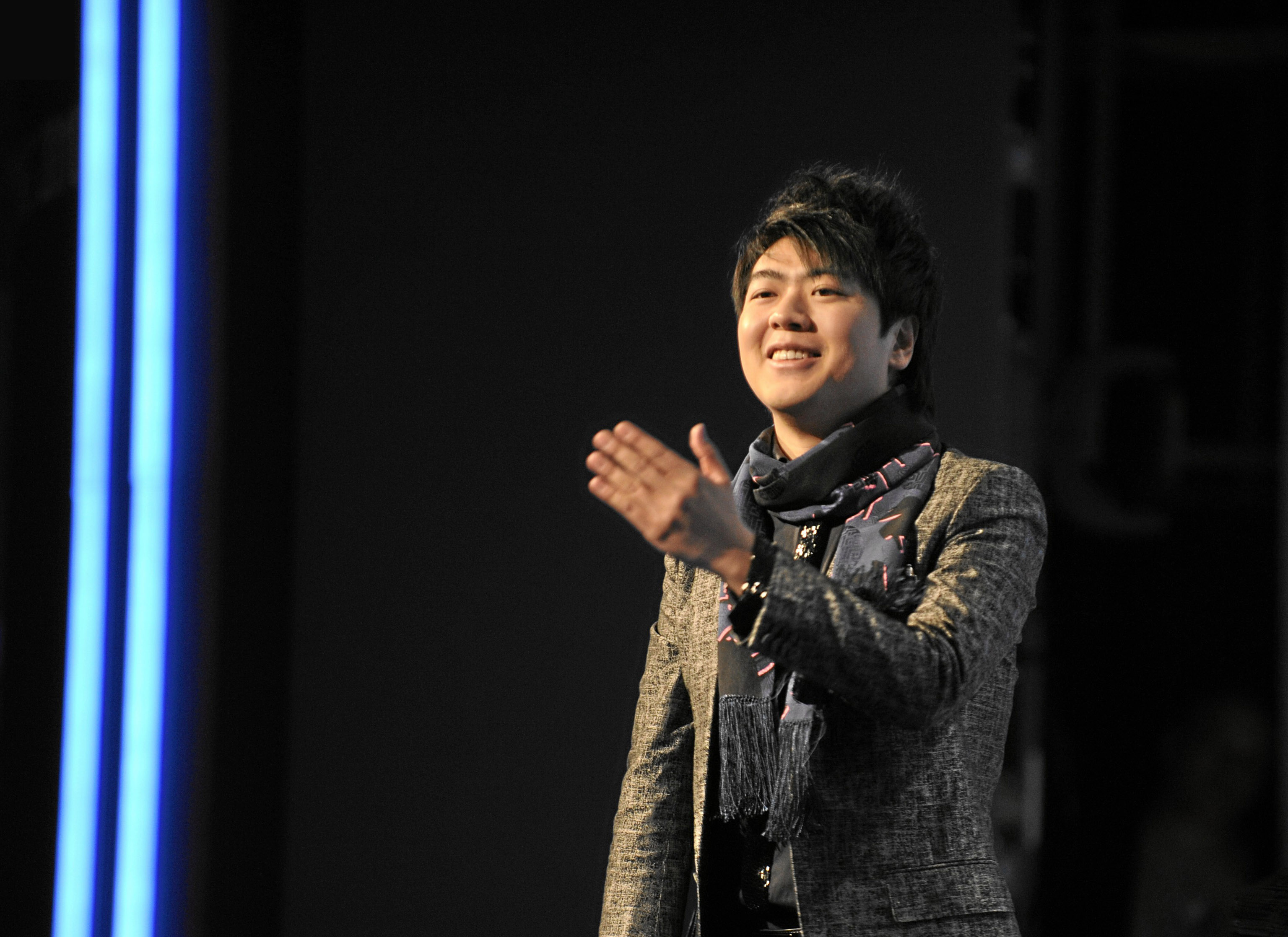The photograph captures a young Asian man standing slightly to the right of the frame, against a predominantly black, grainy background illuminated by two parallel blue LED lights running vertically along the left side. The man, who appears to be in his 20s or early 30s, has dark spiky hair and is smiling warmly as he gestures with his left hand, the palm facing towards his face as if addressing someone out of view. He is dressed in a black and gray textured open coat over a dark button-up shirt, accompanied by a blue scarf adorned with black and pink patterns draped around his neck. The top of his leather belt and a black wristwatch or sleeve cuff are also visible. His overall attire and confident stance suggest a casual yet stylish demeanor, captured in a moment of interaction or expression.